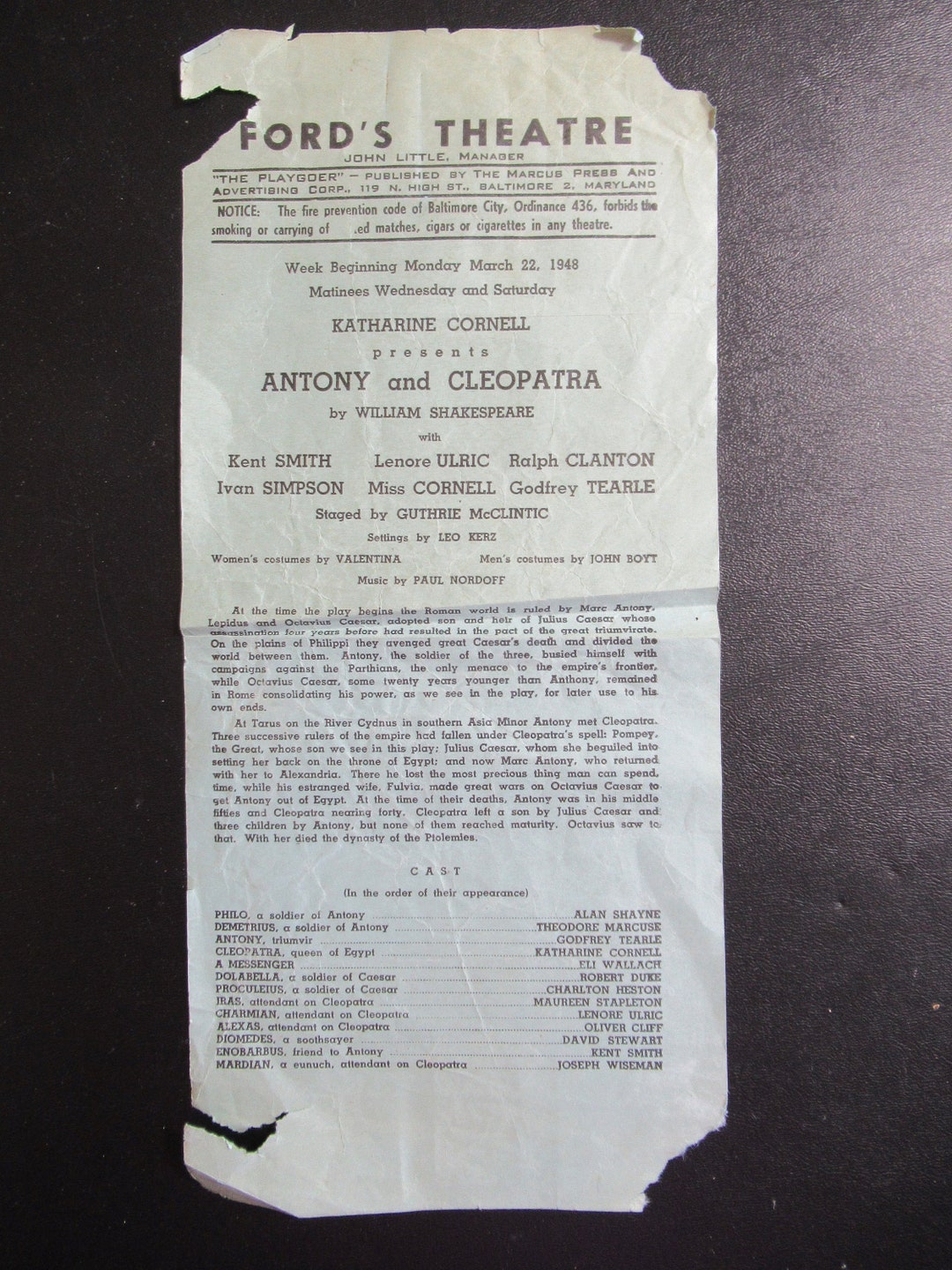In the image, there is an old and worn piece of paper set against a black background. The paper has a noticeable off-white color and is torn and ripped along the edges, with some sections completely missing. At the very top of the paper, "Ford's Theater" is prominently written in black text. Below that, the paper lists "John Little Manager," followed by "The Playgoer," published by the Marcus Press and Advertising Corps with an address provided. Further down, it states "Catherine Cornell Presents Antony and Cleopatra by William Shakespeare." Beneath this title, there are additional paragraphs of information. Towards the bottom, it features a section labeled "cast," listing names such as Kent Smith, Leonard Ulrich, Ralph Clanton, Ivan Simpson, and Godfrey Thiel. The right side of the image has a shiny glare, adding to its aged appearance.